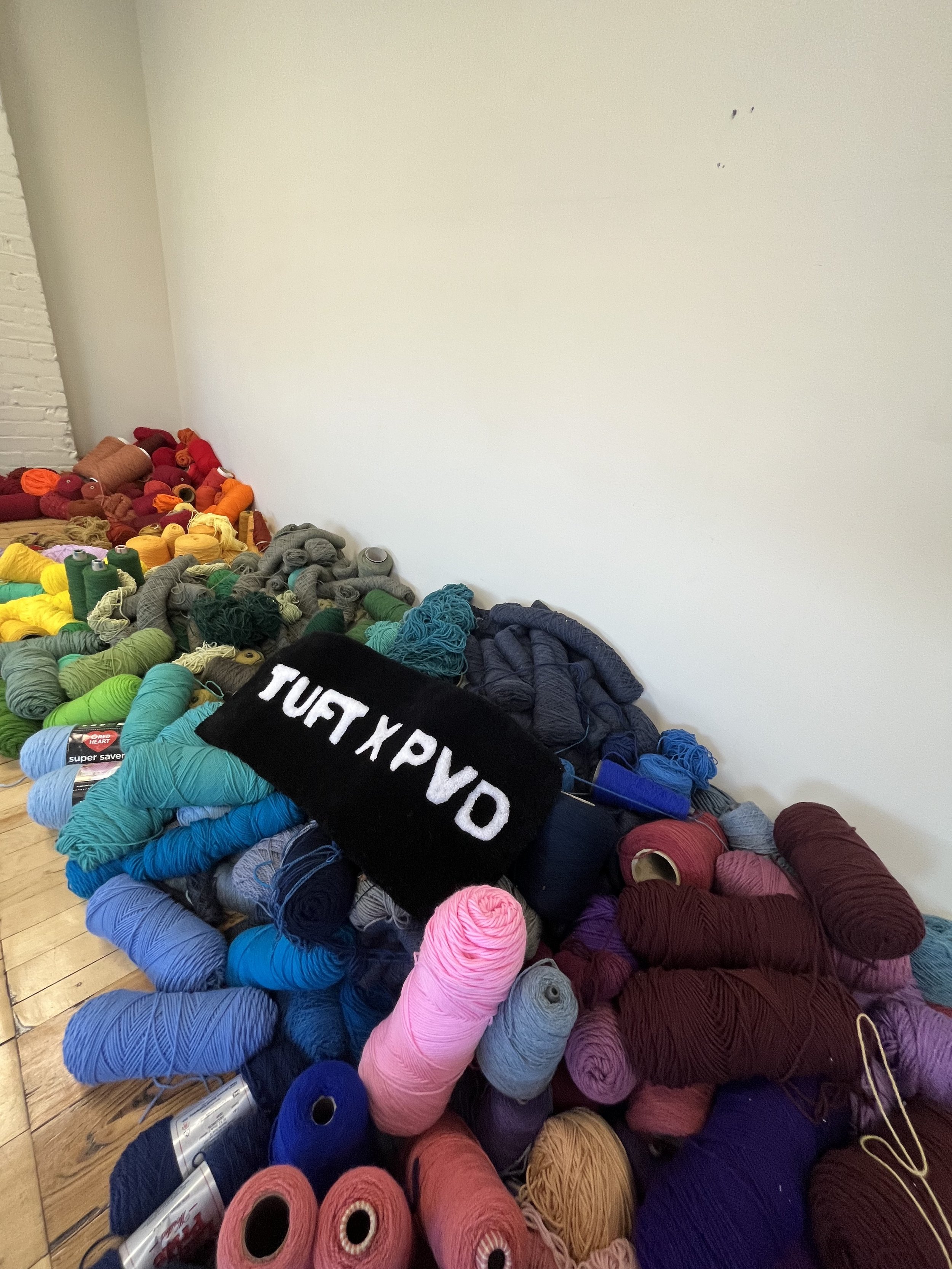This detailed photograph captures an array of vividly colored skeins of yarn, neatly sorted and sprawling across a wooden floor with an off-white wall in the background. The yarns create a striking visual spectrum, beginning with reds and oranges at the far end, transitioning through various shades of yellow, green, teal, and blue, before ending in purples and pinks. Notably, a black piece of fabric, featuring the text "Tuft X PVD" in bold white letters, rests prominently atop this colorful expanse. The "X" likely signifies a collaboration, and "PVD" is presumably the company's name. The careful organization of the yarn, despite the seemingly casual placement, adds an artistic touch to the scene, beautifully highlighting the diversity of colors from vibrant magentas and deep maroons to subtle pastels and rich forest greens. The room appears serene, allowing the dynamic range of yarn colors to take center stage in this thoughtfully composed image.